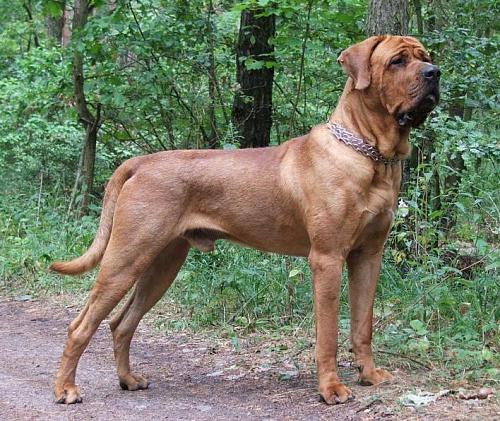The image depicts a large, reddish-brown dog standing alertly on a forest trail, surrounded by trees, grass, and shrubs. The dog has a short but dense coat, resembling a Mastiff, with a strong build and a long tail that curls at the end and hangs down. His head, lifted and turned to the right, reveals wrinkles around his eyes and forehead, along with droopy ears and a black nose. He's wearing a pinch collar and stands with one paw on the dirt path and the other in the shrubbery, looking intently at something off-frame. The overall lighting of the scene is bright but diffused, highlighting the detailed texture of his fur and the natural surroundings.